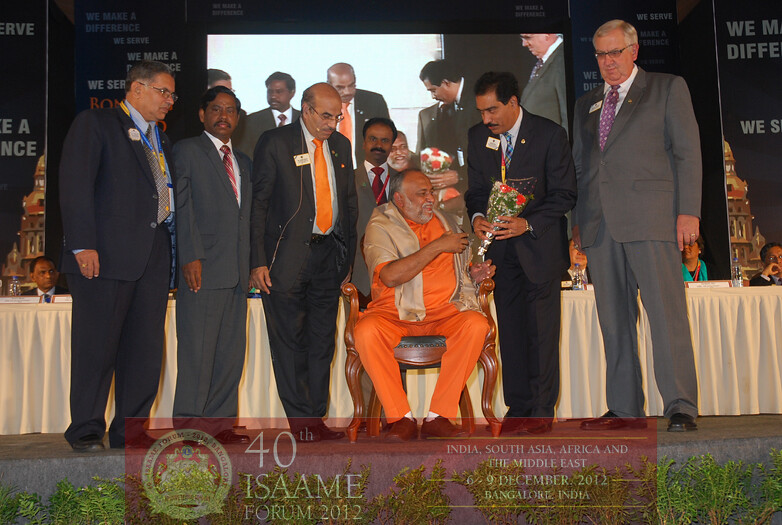In this detailed photograph, we see a distinguished gentleman seated on a wooden stage chair, adorned in vivid orange attire, comprising an orange shirt, orange pants, and a shawl-like covering around his shoulders. His ensemble is completed with white socks and brown shoes. The gentleman is the focal point of the event, as he is being handed a small bouquet of flowers by another man dressed in a dark blue suit and blue tie, positioned to the gentleman's right. 

Surrounding the main figure, there are five other men, three to his left and two to his right, all attired in professional suits and ties. Notably, one man to the gentleman’s left is wearing a black suit paired with an orange tie that matches the seated man's attire, while another man on the far right sports a gray suit with a purple tie.

In the background of the stage, the same scene is projected on a large screen, albeit from a slightly different angle, suggesting a live or delayed feed. A table with a banner is positioned behind the main group, and behind this table are more people, possibly part of the event’s assembly.

The banner prominently displays: "40th ISAME Forum 2012, India, South Asia, Africa, and the Middle East, 6th through the 9th of December 2012, Bangalore, India." This indicates the event is the 40th ISAME Forum held in Bangalore, bringing together delegates from various regions.